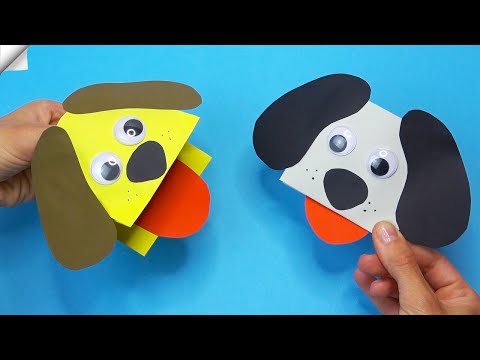In the photograph, a pair of hands hold two colorful, animated dog puppets made from construction paper against a very bright blue background, framed at the top and bottom by black bars. The left hand holds a completed yellow dog puppet with brown ears, large googly eyes, a black nose, and a red tongue sticking out. The right hand grips a similarly styled but incomplete white dog puppet with black ears, a black nose, and a red tongue. This puppet is missing a piece of paper under its mouth, giving it an unfinished appearance. Both puppets have layered ears and dynamic, spin-able eyes, emphasizing their playful and child-friendly design.